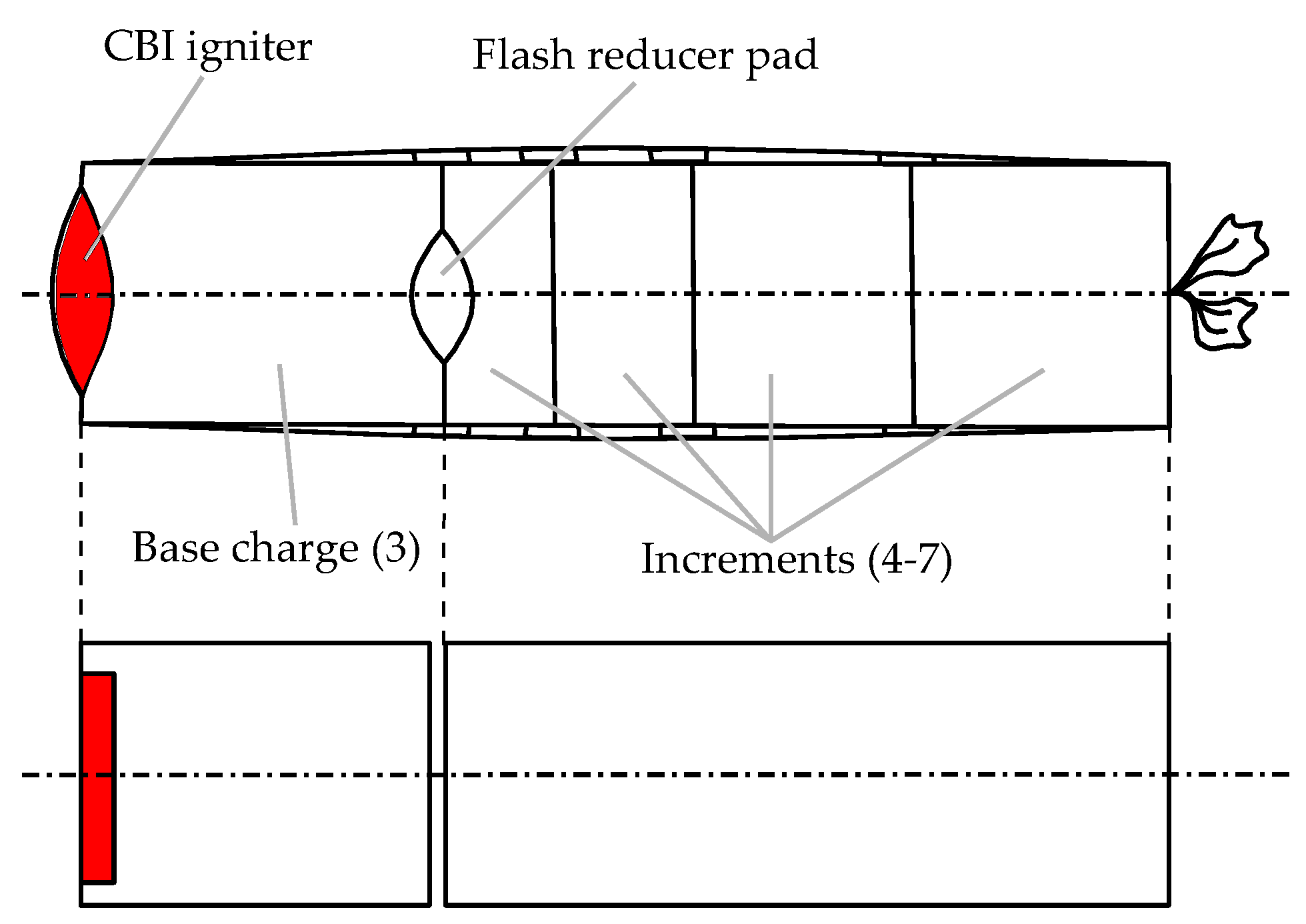The image is a black-and-white illustration resembling a breakdown or map, accompanied by various descriptive labels. It is square-shaped without a distinct border, featuring a detailed layout of multiple sections divided by vertical and horizontal dashed lines. 

At the top left of the image, a red flame-shaped icon labeled "CBI Igniter" is positioned, with a line pointing to it. Adjacent to this, a smaller, black-and-white similar icon is labeled "Flash Reducer Pad." Below these, a large horizontal rectangular section occupies the middle of the image. This rectangle is split into sections by vertical dashed lines, with two leaves hanging off the right side. The left part of the rectangle is labeled "Base Charge (3)," and the right section is labeled "Increments (4-7)." The left side of the rectangle features a vertical red lens-shaped area, contrasting with the primarily white adjacent sections. 

Further down in the image, there is another rectangular section. Its left side includes a vertically standing red rectangular area, divided by another horizontal dashed line in the middle. The detailed diagram is thoroughly annotated with lines pointing to each labeled section, providing a comprehensive explanation of each component.